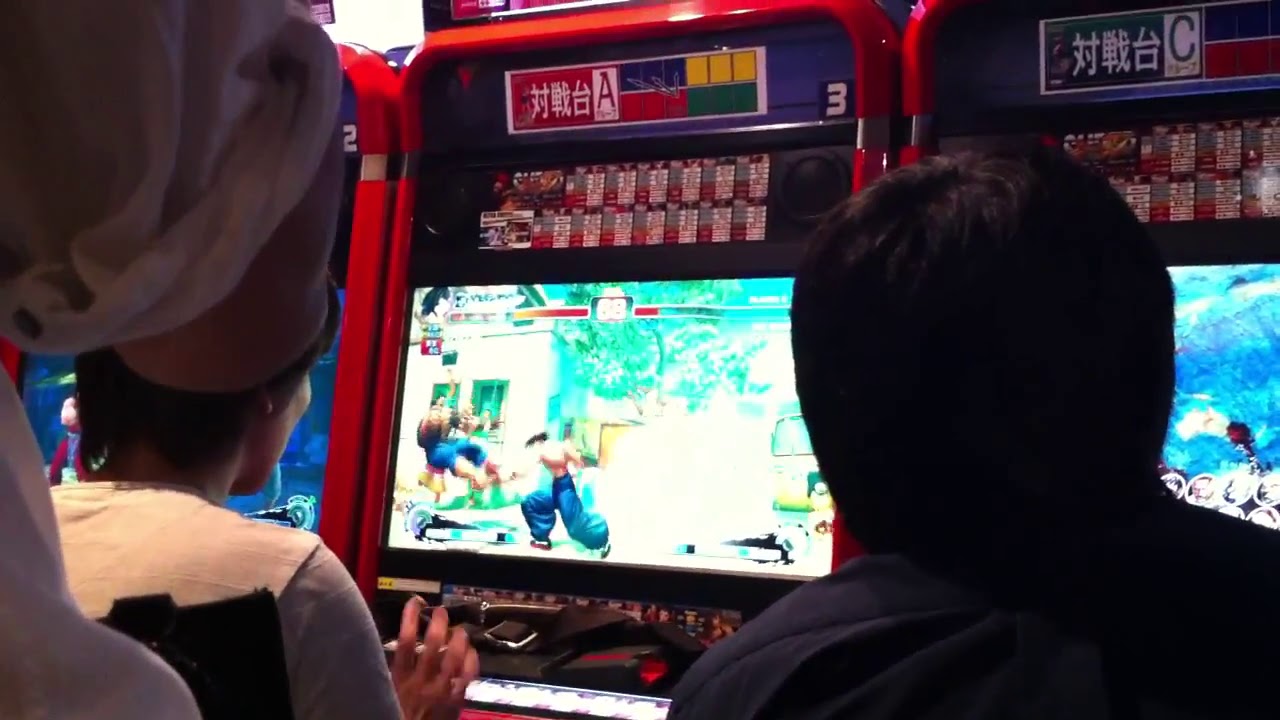In the photograph taken inside an arcade, likely in an Asian country, three people are engaged with tall, red plastic-enclosed arcade machines positioned side by side. The dominant machine, featuring a fighting game reminiscent of Mortal Kombat, displays a dynamic scene where a shirtless character in billowing blue pants delivers a hit to another airborne character clad in blue shorts. At the top of the screen, Asian script is visible, obscuring the game's title. 

The foreground shows three individuals from behind. On the left, a person stands partially visible, donning a white billowy blouse. Below this person, a seated individual with long, straight black hair and a white t-shirt is visible but with their face obscured. To the right, another person with short, straight black hair wears a navy blue or black shirt and is seated, leaving only their head and shoulders visible. Another person, standing nearby to the left, is barely in the shot, noticeable only by their gray sleeve. The immersive environment and positions of the individuals clearly suggest their focus on the vibrant, competitive arcade action.